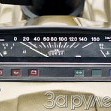The image depicts a small, square dashboard, predominantly in black and gold. At the center of the dashboard is a detailed speedometer, featuring white numerals starting from 0 and increasing by tens up to 160. Surrounding the speedometer are additional gauges and buttons, suggesting a complex and potentially automotive-related instrument panel. The background of the speedometer is black, with all markings and the needle in white, providing clear contrast. Above the speedometer are letters that appear to spell out "3A T Y N E". The visual quality is limited, making it challenging to discern whether the image is a photograph or computer-generated.